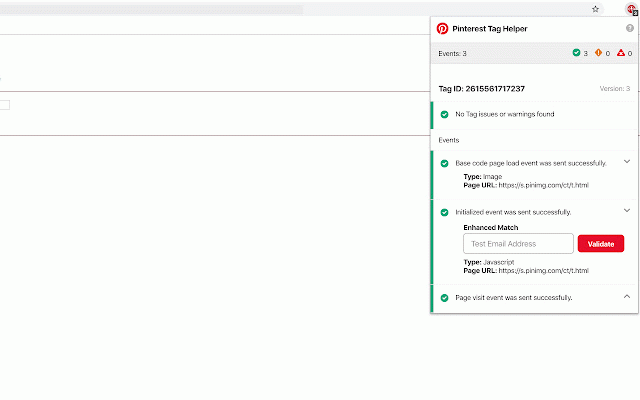In this image, we see a web page interface dedicated to Pinterest Tag Helper. The layout is divided into two sections. The left two-thirds of the image are predominantly blank, only featuring three horizontal lines. On the right third, a header reads "Pinterest Tag Helper" accompanied by a red circle with the recognizable Pinterest 'P' logo. Below this, there's a light gray bar displaying the text "Events 3" in black, followed by three icons: a green circle with a check mark, a red diamond with an exclamation point, and a red triangle with an indistinguishable symbol inside.

Proceeding further down, the text "Tag ID 2615561717237 Version 3" is prominently displayed in black font. The status "No Tag Issues or Warnings Found" follows, highlighted with a green circle and check mark. This is succeeded by the heading "Events," under which several detailed notifications are listed:

1. "Base Code Page Load Event was sent successfully" marked with a green circle and check mark. The event type is Image, but the page URL is too blurry to discern.
2. "Initialized Event was sent successfully," also indicated with a green circle and check mark.
3. The mention of "Enhanced Match" with adjacent white and red rectangles labeled "Test Email Address" and "Validate" respectively.
4. The event type noted as JavaScript, with another page URL that is unreadable.
5. Lastly, "Page Visit Event was sent successfully" is listed at the bottom, paired with a green circle and white check mark.

This comprehensive description encapsulates all the text, icons, and status indicators present in the Pinterest Tag Helper interface.